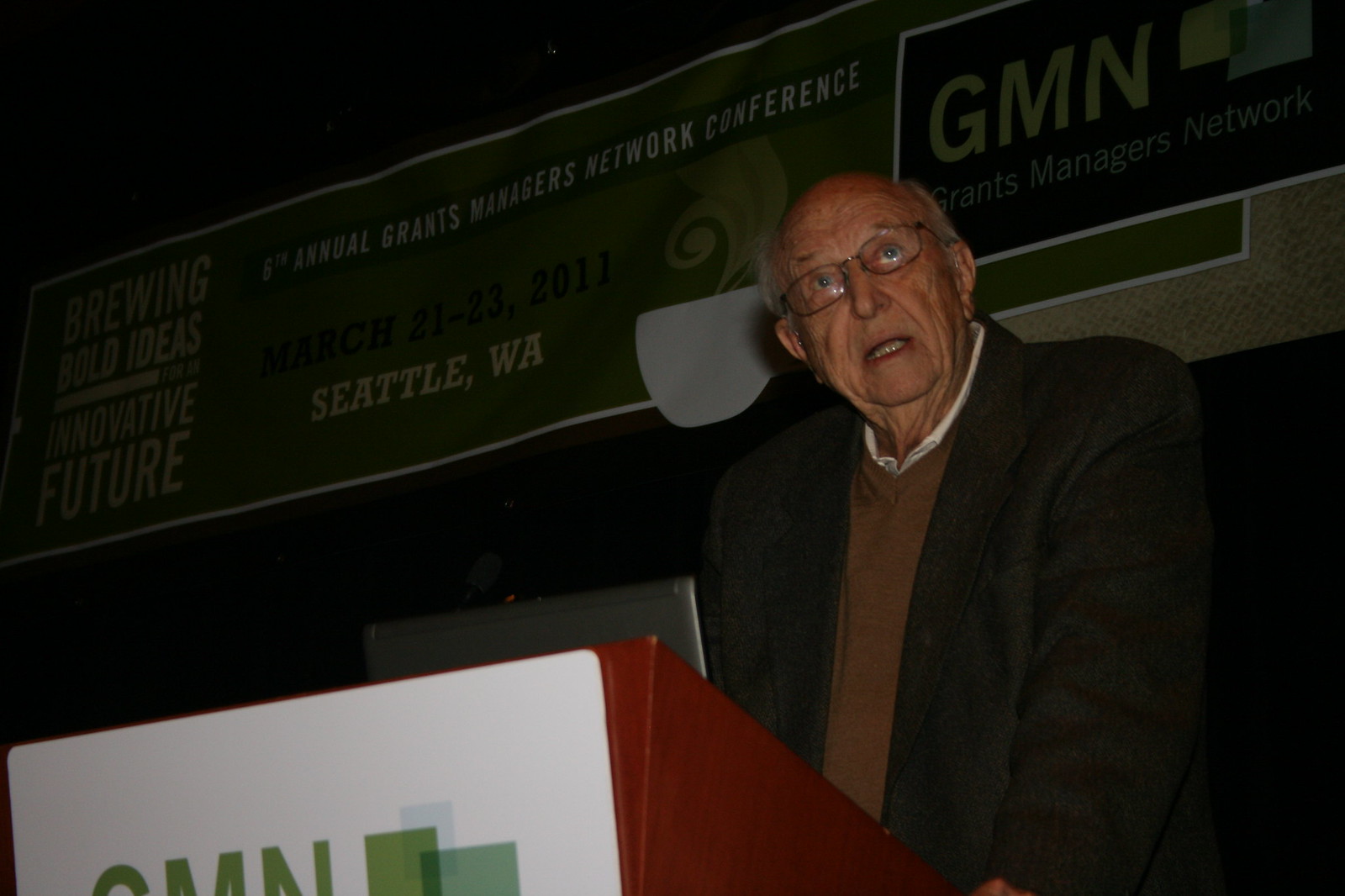In a dimly lit room, an elderly man, likely in his seventies, stands at a wooden podium. He is illuminated by a faint light, which also casts subtle light on a banner behind him. The man, wearing a black blazer over a brown jumper and a white button-down shirt, has gray hair and glasses. His face is deeply wrinkled, and he looks upwards, mouth open, possibly mid-speech. On the front of the podium is a white sign, and he has a laptop or monitor with a visible silver screen in front of him. The green banner behind him, with a white border, reads, "Brewing Bold Ideas for an Innovative Future, 8th Annual Grants Managers Network Conference, March 21 to 23, 2011, Seattle, WA," and features a coffee cup graphic with steam. In the top right corner of the banner is the text "GMN Grants Managers Network."